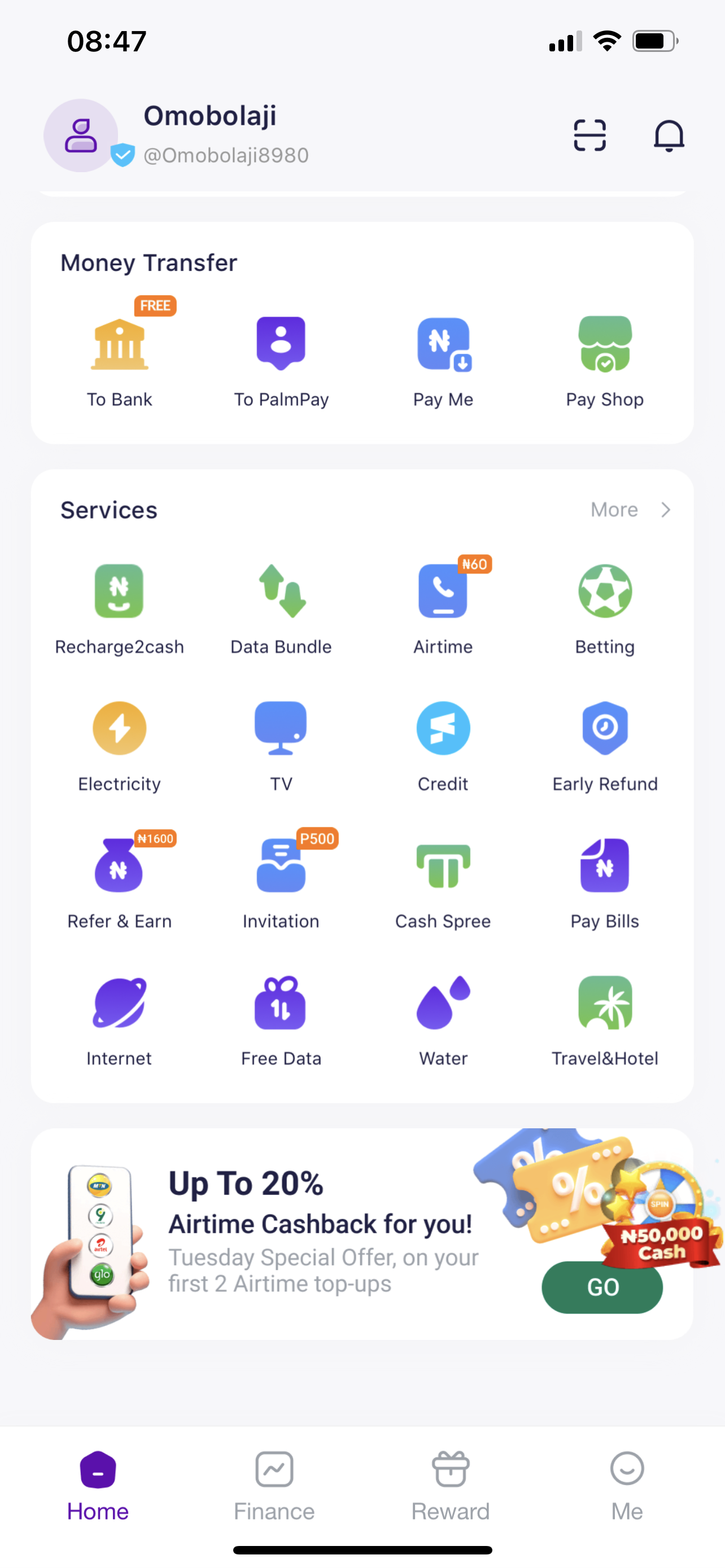The image depicts a cluttered webpage interface with various functionalities and promotional elements. At the top, there's an option to "Flag as inappropriate" displayed in a subtle gray shadow. The time in the upper left corner reads 8:47, while to the right there are icons for energy settings and battery life. 

Prominently featured across the page is the cryptic text "Homage Balaji," with the overall print appearing squished, making readability difficult. Several categories are lined up with corresponding icons, including "Money Transfer," "To Bank," "To Palm Pay," "Pay Me," and "Pay Shop." 

Following this, there's a "Services" line listing options such as "Recharge to Cash," "Data Bundle," "Airtime," and "Betting." The next row features utilities like "Electricity," "TV Credit," and "Early Refund." Below, "Refer and Earn," "Invitation," "Cash Spree," and "Pay Bills" are highlighted. The final line includes "Internet," "Free Data," "Water," "Travel," and "Hotel."

At the bottom, an engaging advertisement showcases a person holding a cellphone. The ad promotes an enticing offer: "Up to 20% Airtime Cashback for You. Tuesday, Special Offer on Your First Two Airtime Top-ups." To the right, there are several marketing icons, including a standout promotion for "$50,000 Cash," next to a vibrant green button labeled "GO" in white letters.